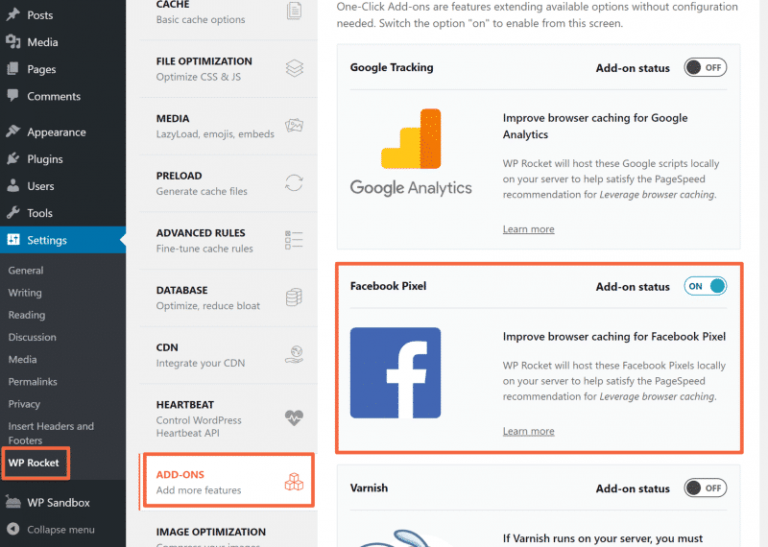The image showcases a busy website interface with numerous elements. On the left, there is a black vertical navigation bar highlighted with blue on the 'Settings' option. This sidebar contains options such as Posts, Media, Pages, Comments, Appearance, Plugins, Users, Tools, and Settings.

Adjacent to the navigation bar is a section with a light gray background. This section contains settings for WP Rocket, outlined in a red box. The WP Rocket settings panel includes options for Cache, File Optimization, Media Preload, Advanced Rules, Database, CDN, Heartbeat, and Add-ons. The 'Advanced Rules' section has a dropdown arrow leading to further settings.

To the right, there is a detailed description about 'One-Click Add-Ons,' featuring options that extend functionality without additional configuration. The add-ons listed include Google Tracking with its status marked as off and Google Analytics emphasizing improved browser caching. The interface features visual elements such as a yellow and orange icon for Google Analytics.

Additionally, there is a 'Facebook Panel' section prominently displayed in the middle, with an on status. It features a blue box with a white 'F' for Facebook and mentions the improvement of browser caching for the Facebook pixel, along with a brief explanation.

Below this, the 'Varnish Add-On' section is mentioned with its status marked as off. The interface details are cut off at this point, leaving the following elements of the website unspecified.